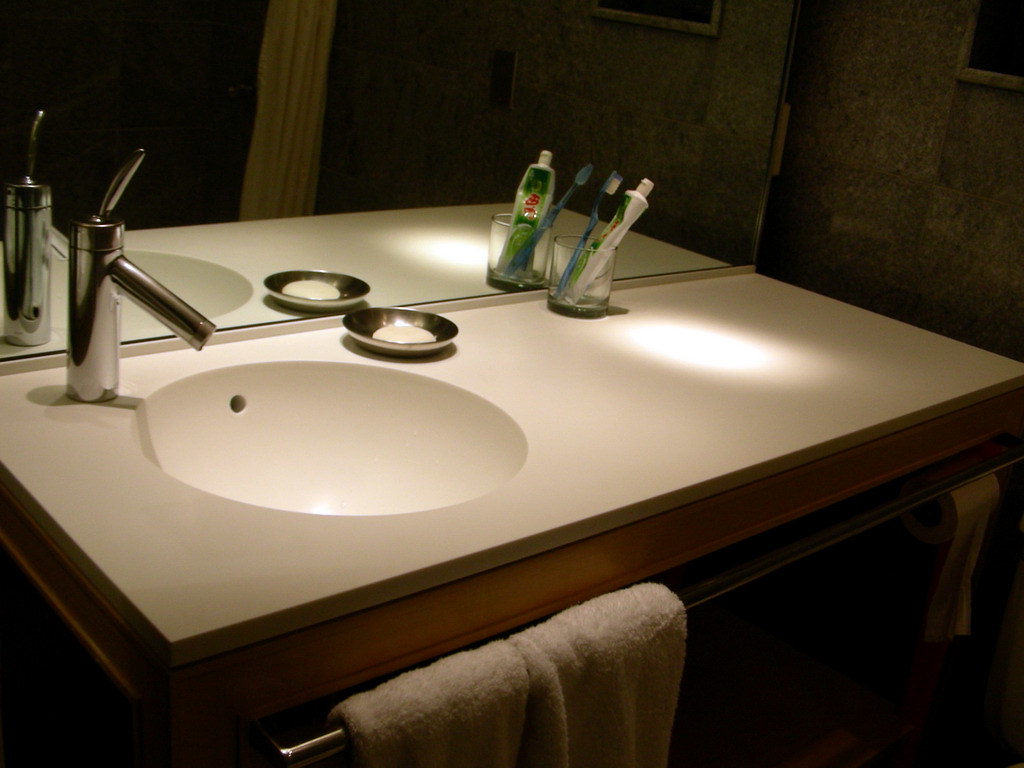The image showcases the sink area of a bathroom featuring a substantial mirror that reflects the sink and adjoining items. At the forefront is a sleek silver faucet set against a pristine white countertop and sink basin. Resting on the counter is a silver soap dish holding a white bar of soap. Adjacent to the soap dish is a glass cup that contains a bottle of toothpaste and a blue toothbrush. Positioned in front of the counter, a towel rack holds two neatly arranged towels, with a roll of toilet paper hanging loosely nearby. The background reveals a wall adorned with gray tiles and hints of a windowsill. The overall lighting in the image is dim, with the main illumination focused on the counter area, leaving the rest of the scene in relative shadow.